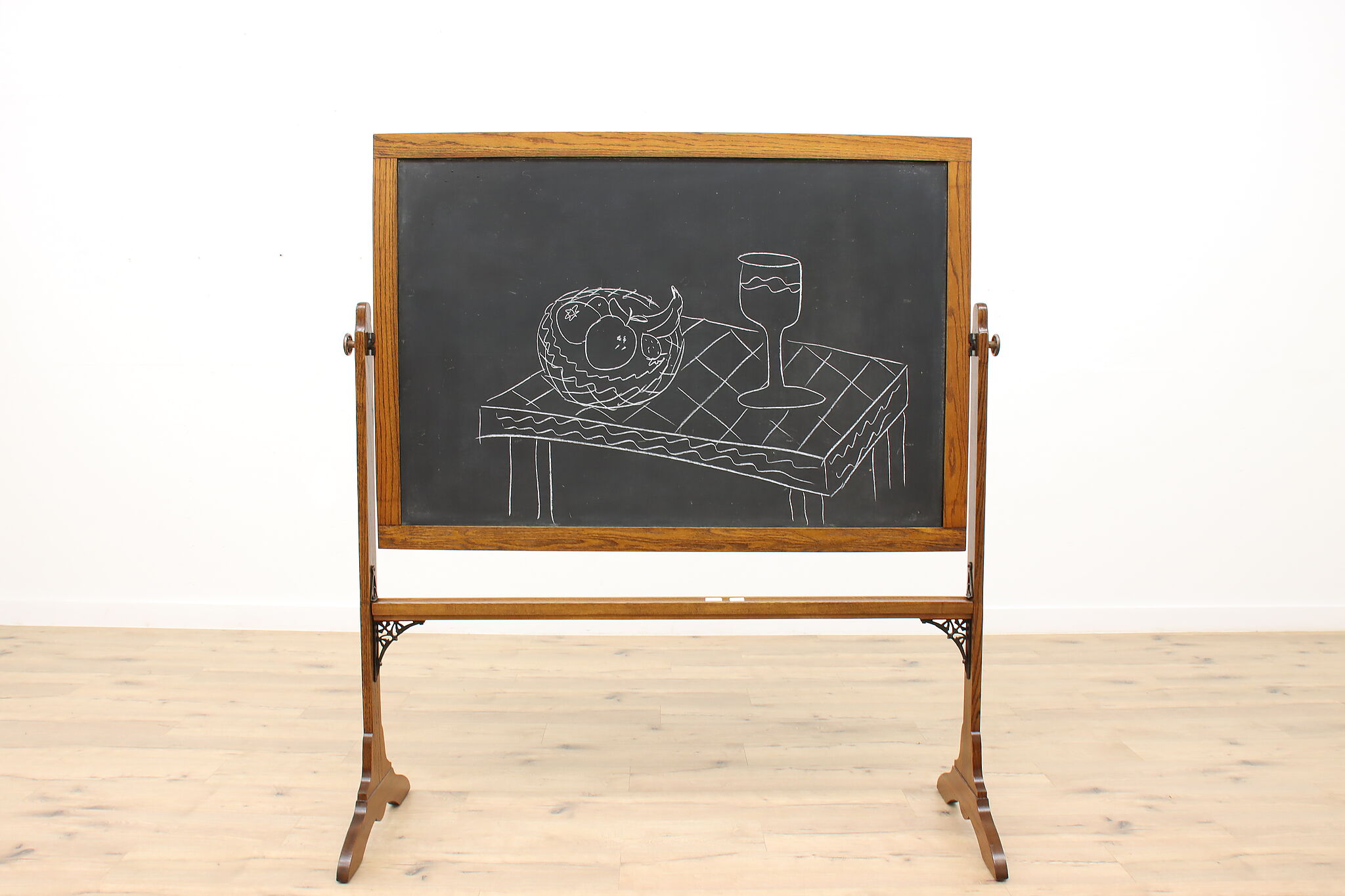In a brightly lit room with pristine white walls and light beige wooden floors stands a vintage-style chalkboard framed in rich brown wood. The rectangular chalkboard, black in color, is mounted on an easel-like structure that allows it to swivel. This old-school blackboard features metal curves on its frame and stands on sturdy legs connected by a horizontal support. The chalkboard displays a simplistic, white chalk drawing depicting a thick, grid-patterned table. On the table rests a goblet-like glass of beverage and a round basket filled with fruit, including bananas, tomatoes, and strawberries. The entire scene, though quickly sketched, brings a nostalgic charm to the minimalist setting.